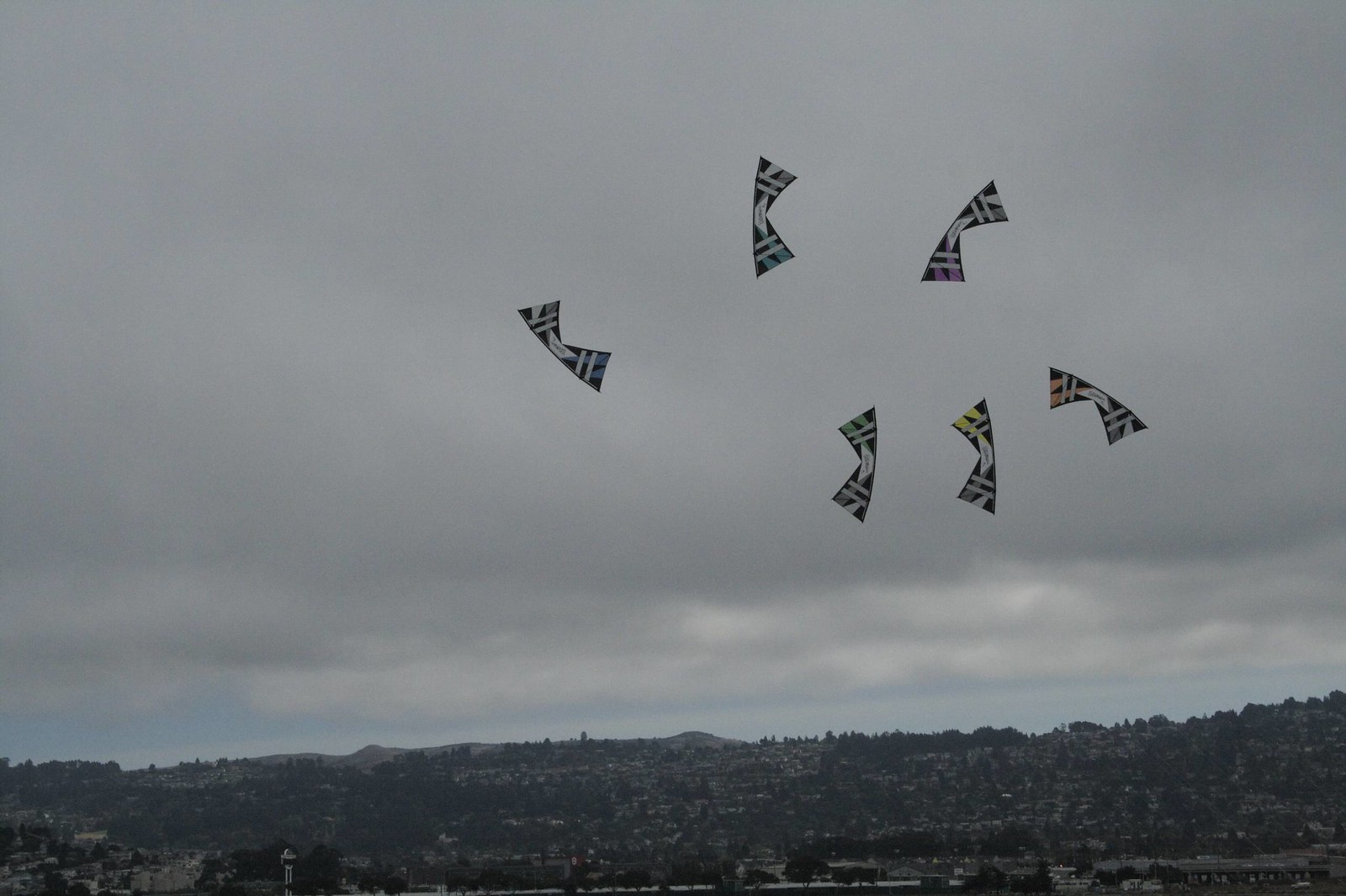This photograph captures a wide shot of a cloudy, gray afternoon sky, dominated by uniform, misty clouds that almost completely obscure the blue of the sky. Beneath the cloud cover, a hilly and forested horizon line can be seen, indicating a rural area with sparse buildings, suggesting the outskirts of a city rather than its densely built center. Six uniquely shaped, wing-like kites, predominantly black with specks of yellow and white, are flying in a semi-circle pattern across the sky, creating a striking contrast against the overcast backdrop. The scene provides a serene yet mysterious atmosphere, emphasizing the dark silhouettes of the kites against the gloomy clouds.